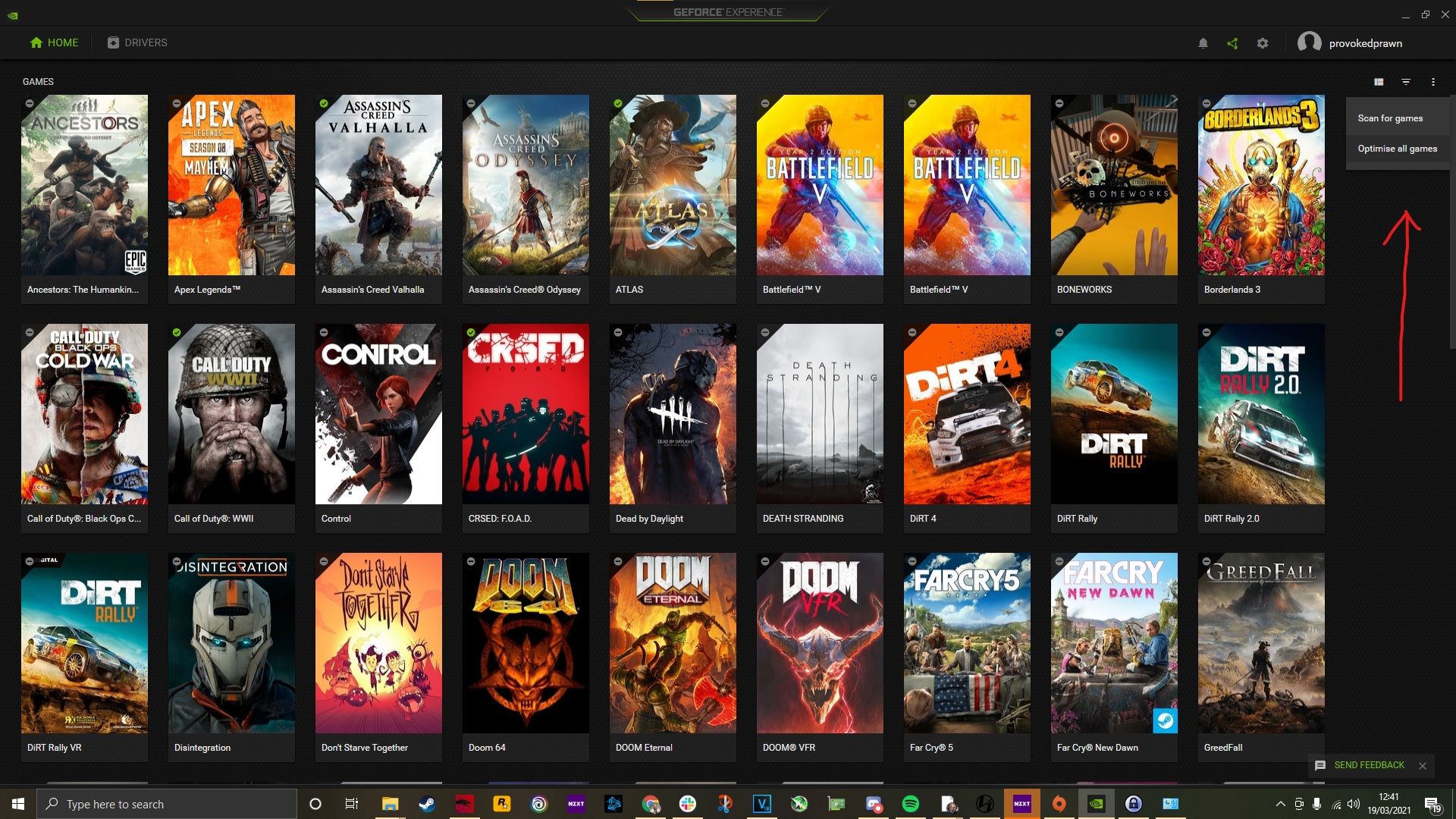The image is a screenshot of a website dedicated to video games. On the top-left corner, there's a green icon of a house accompanied by the word "Home". Immediately to the right, there's a right-facing arrow inside a gray box followed by the word "Drivers" in gray. Below this section, on the left, the word "Games" is prominently displayed in white.

The main content area features three rows, each containing nine video game titles. 

**Top Row:**
1. Ancestors
2. Apex Season of Mayhem
3. Assassin's Creed Valhalla
4. Assassin's Creed Odyssey
5. Atlas
6. Battlefield V
7. Battlefield V (repeated)
8. Boneworks
9. Borderlands 3

**Middle Row:**
1. Call of Duty: Black Ops Cold War
2. Call of Duty: World War II
3. Control
4. C.R.S.E.D.
5. Dead by Daylight
6. Death Stranding
7. Dirt 4
8. Dirt Rally
9. Dirt Rally 2.0

**Bottom Row:**
1. Dirt Rally (repeated from the middle row)
2. Disintegration
3. Don't Starve Together
4. Doom 64
5. Doom Eternal
6. Doom VFR
7. Far Cry 5
8. Far Cry New Dawn
9. Greedfall

On the right-hand side, there are two buttons embedded in a background area. One button is labeled "Scan for Genres" and the other "Optimize All Games". Below these buttons, an upward-facing red arrow points towards them.

This detailed orientation provides a comprehensive view of the website’s layout and some of the video games it features.